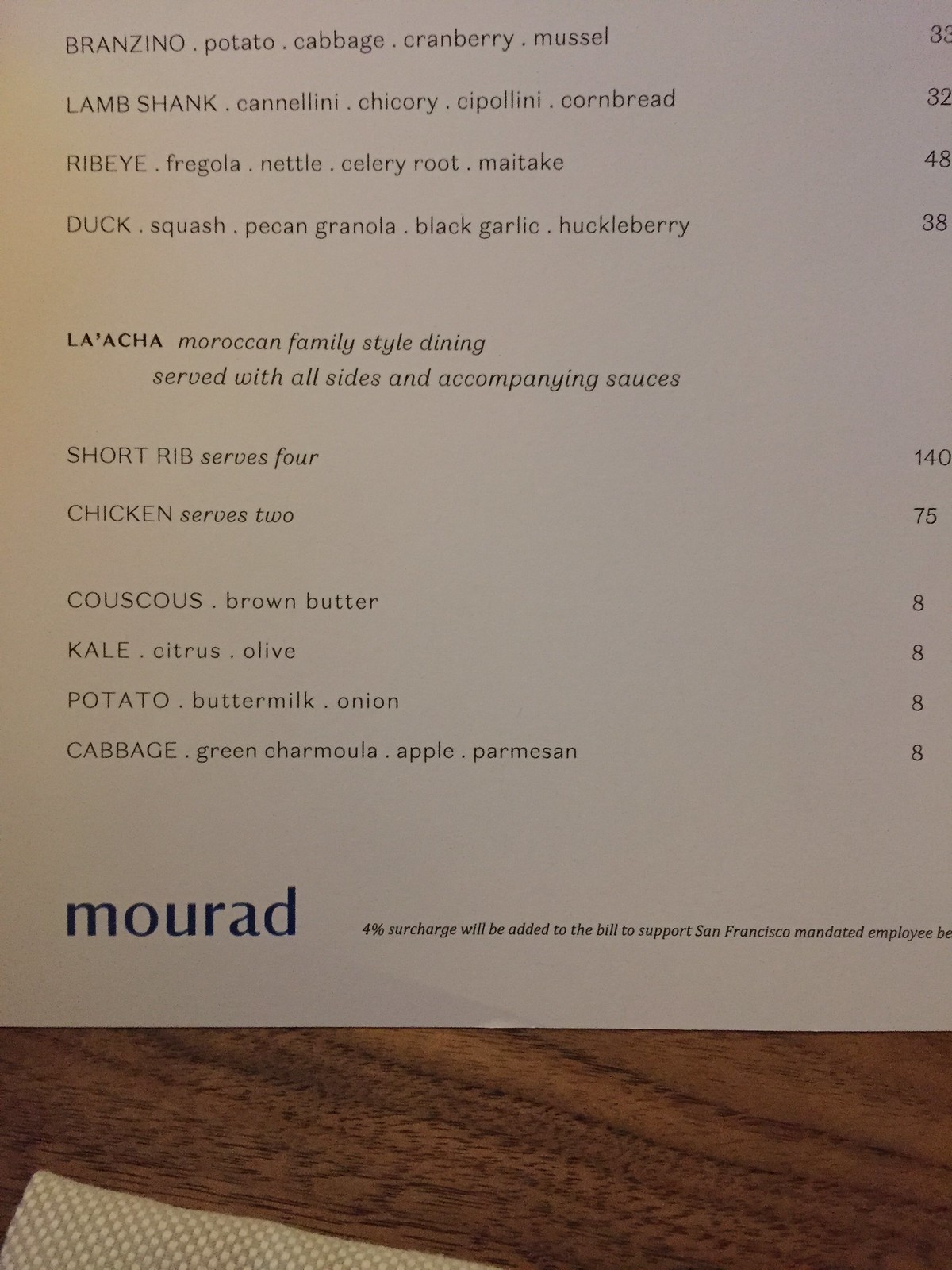This image is a close-up shot of a menu page, displayed on a wood-grained table. The menu appears to be printed on white paper. In the bottom left corner, the name "Mourad" is printed clearly, which is likely the name of the restaurant or hotel. Below this, in very small text, it mentions that a "four percent surcharge will be added to the bill to support San Francisco mandated employee" but the text is partially cut off and incomplete.

The rest of the menu features finely typed black text listing various dishes and their accompanying ingredients. Some highlighted items include:

- **Branzino**: paired with potato, cabbage, cranberry, and mussel.
- **Lamb Shank**: described with cannellini, chicory, cipollini, and cornbread.
- **Duck**: served with squash, pecan granola, black garlic, and huckleberry.
- **Ribeye**: though specific accompanying ingredients are not listed in this excerpt.
- **Short Rib**: accompanying ingredients are not detailed in this excerpt.
- **Chicken**: accompanying ingredients are not specified in this excerpt.
- **Couscous**: likely a side or an ingredient, exact pairings not detailed here.
- **Kale**: possibly a side dish.
- **Potato and Cabbage**: may be accompaniments or components of other dishes.

Overall, the menu page is detailed with various gourmet offerings and emphasizes a sophisticated dining experience.